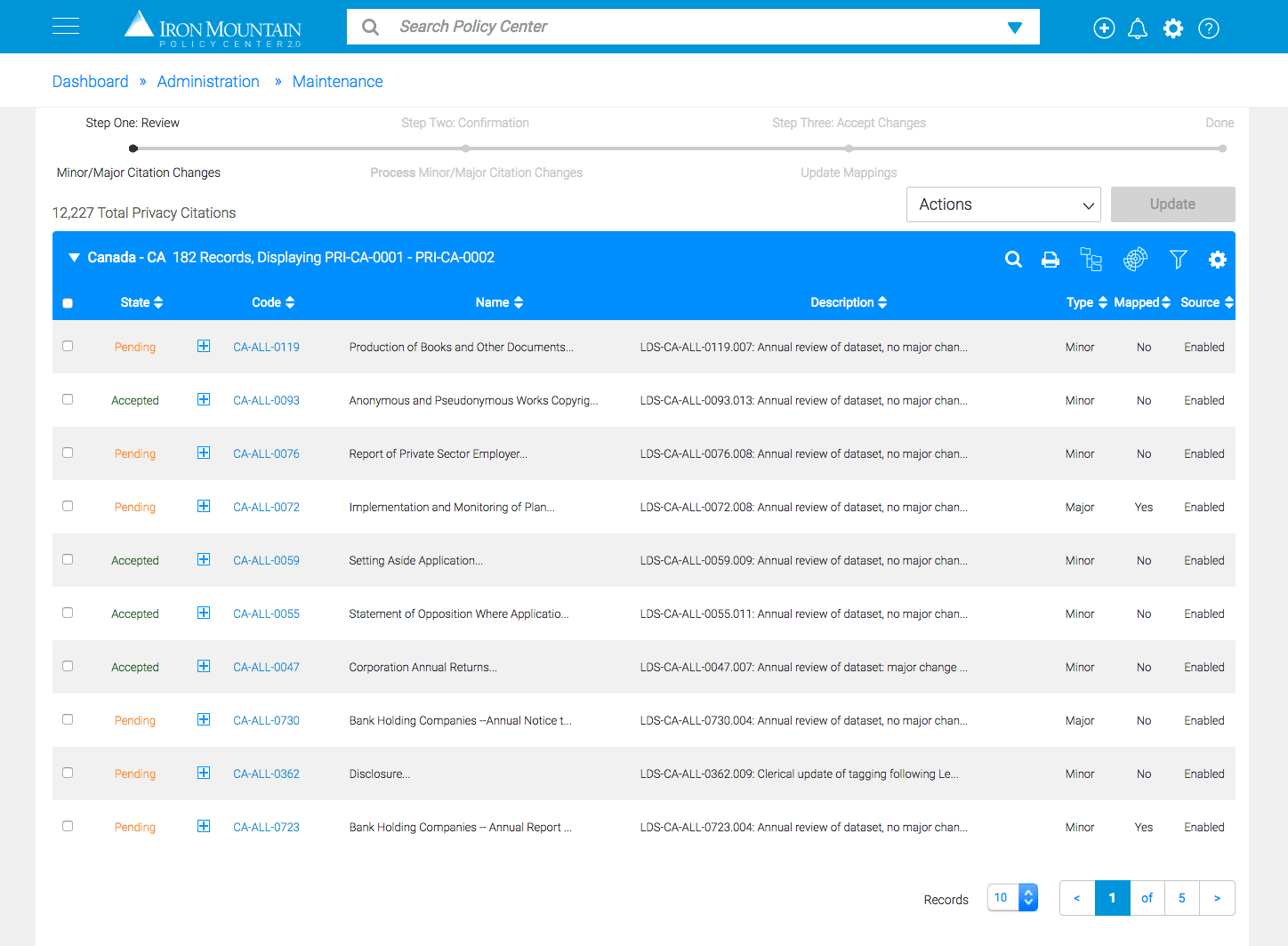This screenshot depicts the Iron Mountain Policy Center 2.0 website. At the top of the screen, a blue banner is prominently displayed. On the left-hand side of this banner, three horizontal lines are visible, which likely lead to a drop-down menu of various options or categories. Centrally placed on the banner is the Iron Mountain Policy Center logo, resembling a triangle or pyramid. Next to the logo, the text "IRON MOUNTAIN" is written in capitalized, white letters, followed by "Policy Center 2.0" in smaller text beneath it.

To the right of the logo, a search bar is provided with the placeholder text "Search Policy Center" and an accompanying down arrow for additional options. Further to the right, icons for a plus sign in a circle, a notification bell, settings represented by a gear wheel, and a help button depicted as a question mark in a circle are aligned.

Below the banner, the main section of the screen displays the header "DATS Forward Administration and Maintenance." Under this header, a list of various records is shown, categorized as either pending or accepted. This list includes:

- Production of Books and Other Documents
- Anonymous and Pseudonym Works Copyright
- Report of Private Sector Employer
- Implementation and Monitoring of Plans
- Setting Aside Application
- Statement of Opposition to Your Application
- Corporation Annual Returns
- Bankholding Companies Annual Notice, Disclosure
- Bankholding Companies Annual Report